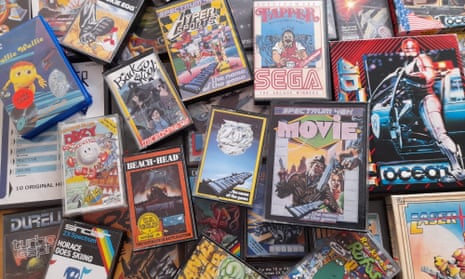The image is a small, horizontally aligned rectangular picture featuring a cluttered collection of video game and movie cases haphazardly stacked and piled on a flat surface. There are over twenty rectangular covers, some vertically aligned while others are stacked on top of each other. The cases come in various colors, including blue and yellow.

Prominently visible titles include "Tapper" by Sega, "Hyper Sports," "Horace Goes Skiing," "Durelli," and "Beachhead." One game in the upper right corner shows a person stepping out of a vehicle with the title "Ocean" beneath them. Another towards the middle right displays a gun on the cover with the title "Movie." In the lower right corner, there's a case labeled "Laser." The overall scene is a chaotic mix of different video game and movie cases, creating a vibrant and somewhat disorganized visual array.